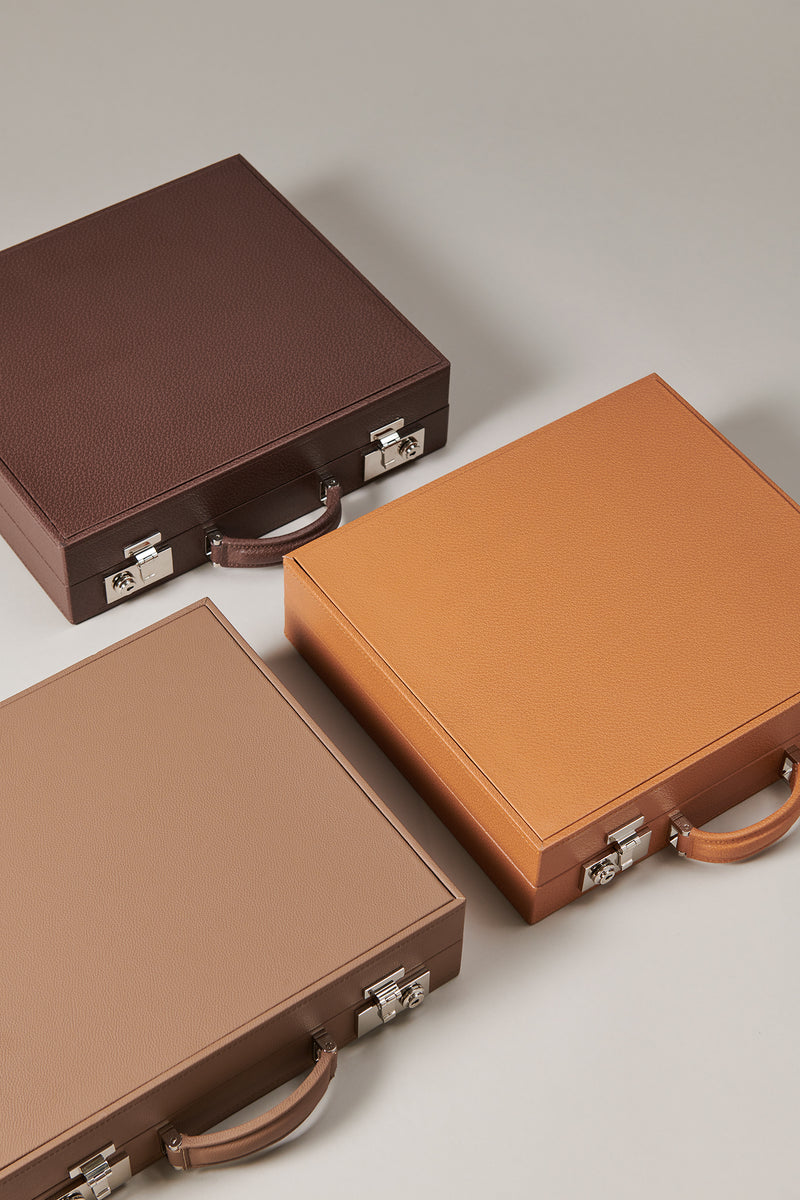This photographic image, taken indoors, captures three briefcases arranged diagonally from the bottom left to the top right, casting shadows onto a gray surface beneath them. The briefcases appear to be made of leather and share similar designs, each equipped with a handle and two metallic latches and keyholes. The briefcase positioned at the top is a dark chocolate brown, slightly smaller than the others, likely due to perspective, with a matching dark brown handle. The briefcase on the bottom left is a very light brown, almost tan, with a similar light brown handle and silver latches. The briefcase on the bottom right is a lighter brown with a hint of orange, featuring the same metallic hardware. There is no text in the image, and part of each briefcase is slightly cut off by the frame.